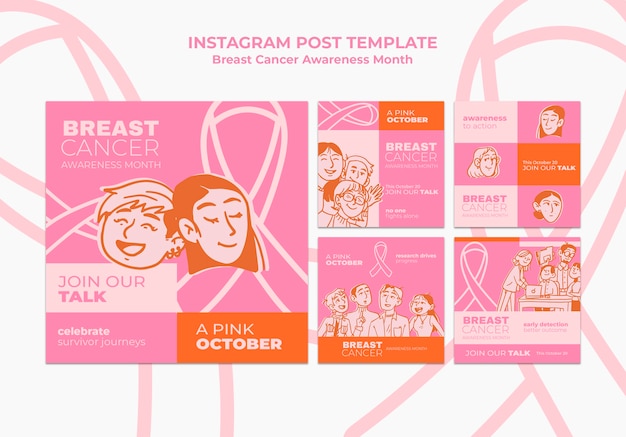The image appears to be a webpage or a digital design template for creating Instagram posts, specifically aimed at promoting Breast Cancer Awareness Month. The primary background color is pink, reinforcing the theme of breast cancer awareness. 

At the top in large, bold, pink text, it reads "Instagram Post Template," indicating its purpose. Below, a prominent section highlights "Breast Cancer Awareness Month" written in pink and red on a pink background. This main section features a large square illustration of two cartoon-like women's faces, emphasizing a cheerful and supportive atmosphere. Accompanying text reads, "Join Our Talk. Celebrate Survivor Journeys. A Pink October."

Adjacent to this main illustration, various other template options are displayed. Each template retains the central theme but offers different design layouts. For example, a smaller square template also has "A Pink October" above "Breast Cancer Awareness Month," and text encouraging participation in talks. It similarly incorporates cartoon illustrations of women, although the characters and layouts vary.

Beneath these, additional templates present the same essential information but with diverse arrangements and different cartoon figures. Each variation maintains a consistent message focused on promoting participation and celebrating survivors during Breast Cancer Awareness Month.